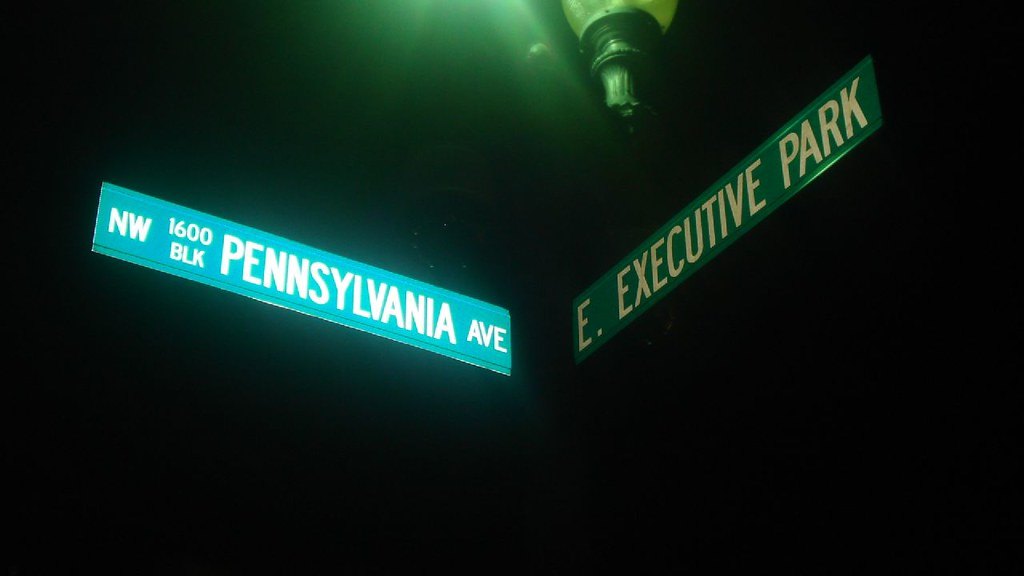In this night-time image, the scene is dominated by two distinct street signs set against a black backdrop, with a nearby lamppost faintly illuminated. The primary signpost, located near the famous 1600 Pennsylvania Avenue, is bathed in a yellowish-green light, giving its typically green and white surface a turquoise tint. This sign features the text "NW 1600 BLK Pennsylvania AVE," clearly indicating its association with the White House's iconic address. Adjacent to this, another street sign remains lit up in its original green hue, reading "E. Executive Park" in uppercase white letters. The light source suffusing this scene appears to originate from another street lamp, which isn't visible, but casts an ambient glow, leaving everything besides the signs and the top portion of the lamppost in darkness.